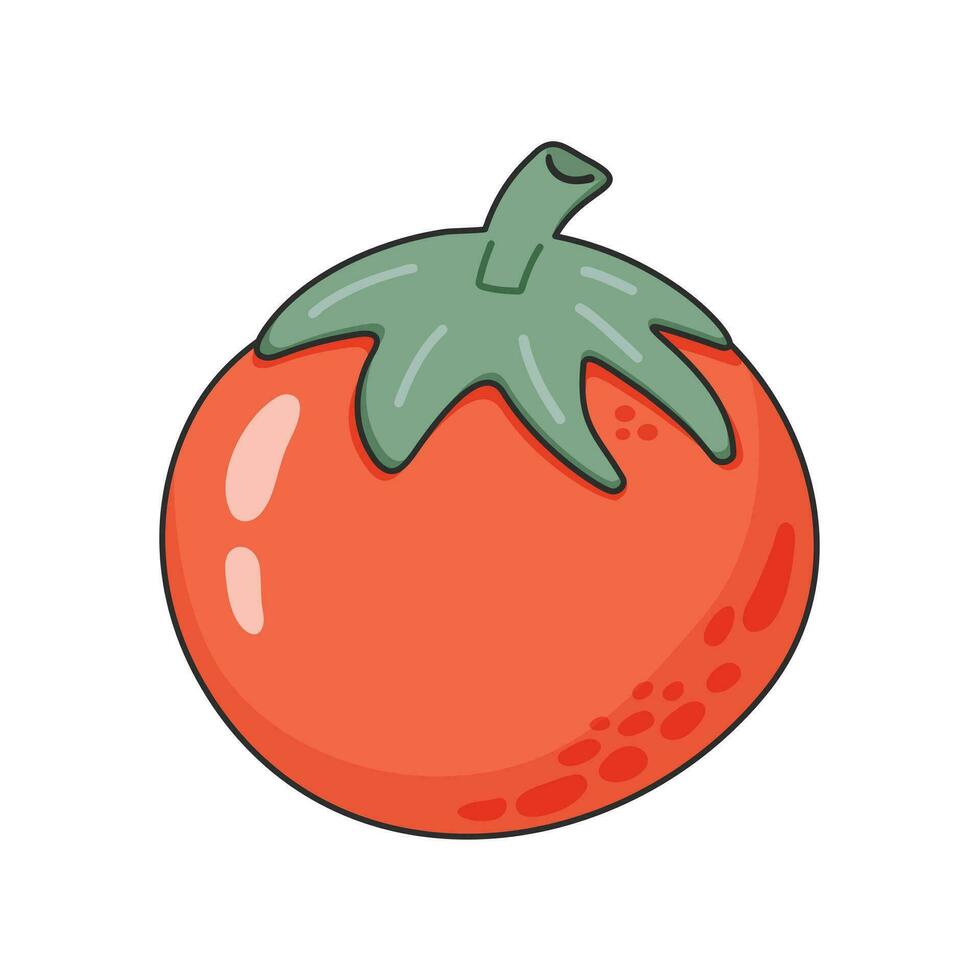This image features a cartoonish drawing of a tomato set against a plain white background. The tomato is predominantly a reddish-orange color with a distinct green stem and leaf structure atop it. The stem comprises four leaves with lighter green lines accentuating the texture, resembling a hand with four fingers. The tomato itself is round, outlined in black, and adorned with various shading and highlights. Notably, the bottom right section shows darker red shadows interspersed with about ten smaller oval-shaped spots, while the top left area displays two lighter red or pink ovals suggesting a reflection of light. The overall art style is reminiscent of Scott Pilgrim's comic book aesthetics, characterized by its 2D, simplistic yet expressive design.